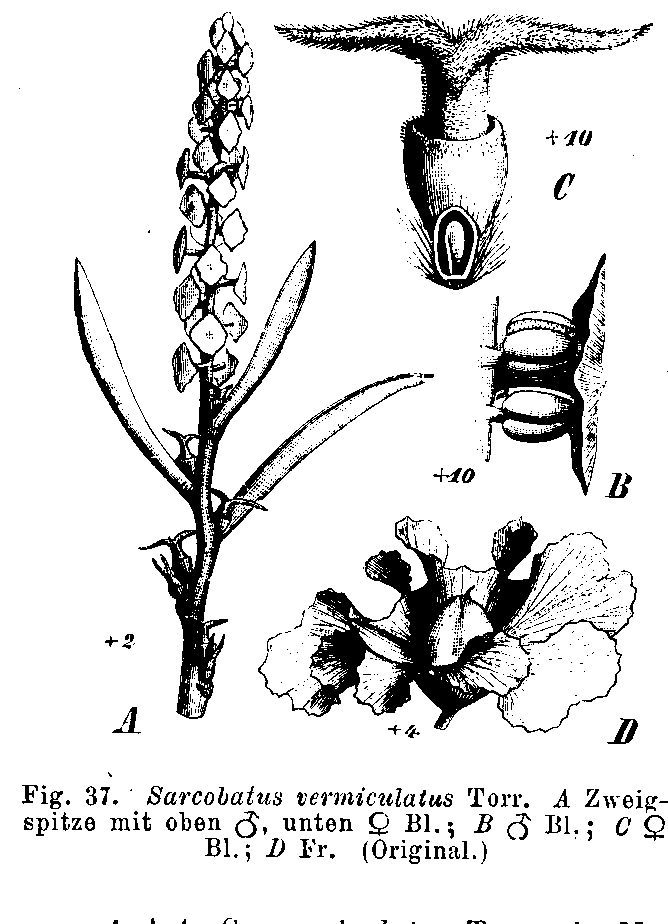The image depicts a black and white scientific infographic labeled "Figure 3-7 Sarcobatus Verniculatus TORR." 
 At the top, there are several annotated illustrations of various flower parts, each labeled with letters A, B, C, and D. 
Item A resembles a long flower stem, item B features two bulbous shapes with a petal-like structure to the side,
item C appears as a seedling, and item D depicts an opened flower petal. The image includes zoom levels indicated as +2, +4, +10, and +10, suggesting varying degrees of magnification. Additionally, detailed notes and numerical annotations are seen throughout, emphasizing the scientific nature of the diagram. The description also contains an assortment of abbreviations and potentially foreign words such as "Sexpitze Mitte Oben Unten," "B-L," "B-B-L," "C-B-L-D-F-R," and "Original" that are likely part of the labeling system used for categorization or identification within the graphic.